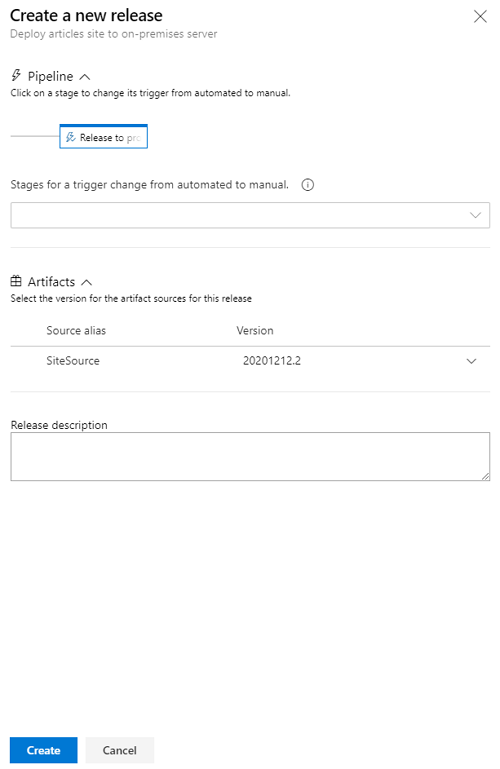In the image, we have a user interface displayed on a white background. At the top, there is a header titled "Create a New Release" with a close (X) button situated on the right. Below the header, highlighted in light blue, is the text "Deploy article site to on-premises server."

Next to this, there is a "Pipeline" section featuring a lightning bolt icon and an upward arrow. Adjacent to this, there's an instructional text: "Click on a stage to change its trigger from automated to manual."

A horizontal gray line separates this section from the subsequent elements. Below the divider, there is a blue-bordered box with a white interior. This box is labeled "Release to," accompanied by a small icon and text indicating "stages for a trigger change from automated to manual." There is also a small circle with an information (i) icon.

Next to the blue box, there is a drop-down menu icon represented by a downward arrow. Under this menu, there is a square divided into four parts labeled "Artifacts." An upward arrow points to this section with an accompanying instruction: "Select the version for the artifact sources for this release."

Details within this section include "Source alias" and "Version." Following this, there is a line separating additional information: "Site source: 2020-12-12," followed by another downward arrow. Below this, a section marked "Release Description" features a large white text box outlined in gray.

In the lower right-hand corner, two small lines cross the corner, and at the very bottom, two buttons are visible: a blue "Create" button and a gray "Cancel" button.